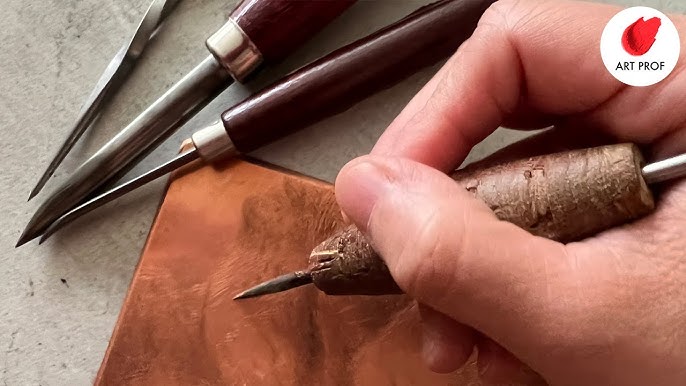In this extreme close-up image, a fair-skinned person’s hand is prominently featured, gripping a pointed leather working tool designed for intricate carving. The thicker base of the tool aids in a firm grip, suggesting precision in the task at hand. Their fingers hover above a copper plate, poised to engrave with the sharp-tip implement. Adjacent to the hand, three additional tools are laid out on what appears to be a marble surface. Each tool varies slightly: one has a dark wooden handle with a thin, pointed metal tip; another features a gold circular base and a thicker pointed end; the third implement has a twisted metal design. In the upper right corner of the image, a white circular emblem with a textured red paint smear reads "Art Prof," indicating a possible affiliation with an art tutorial or resource.